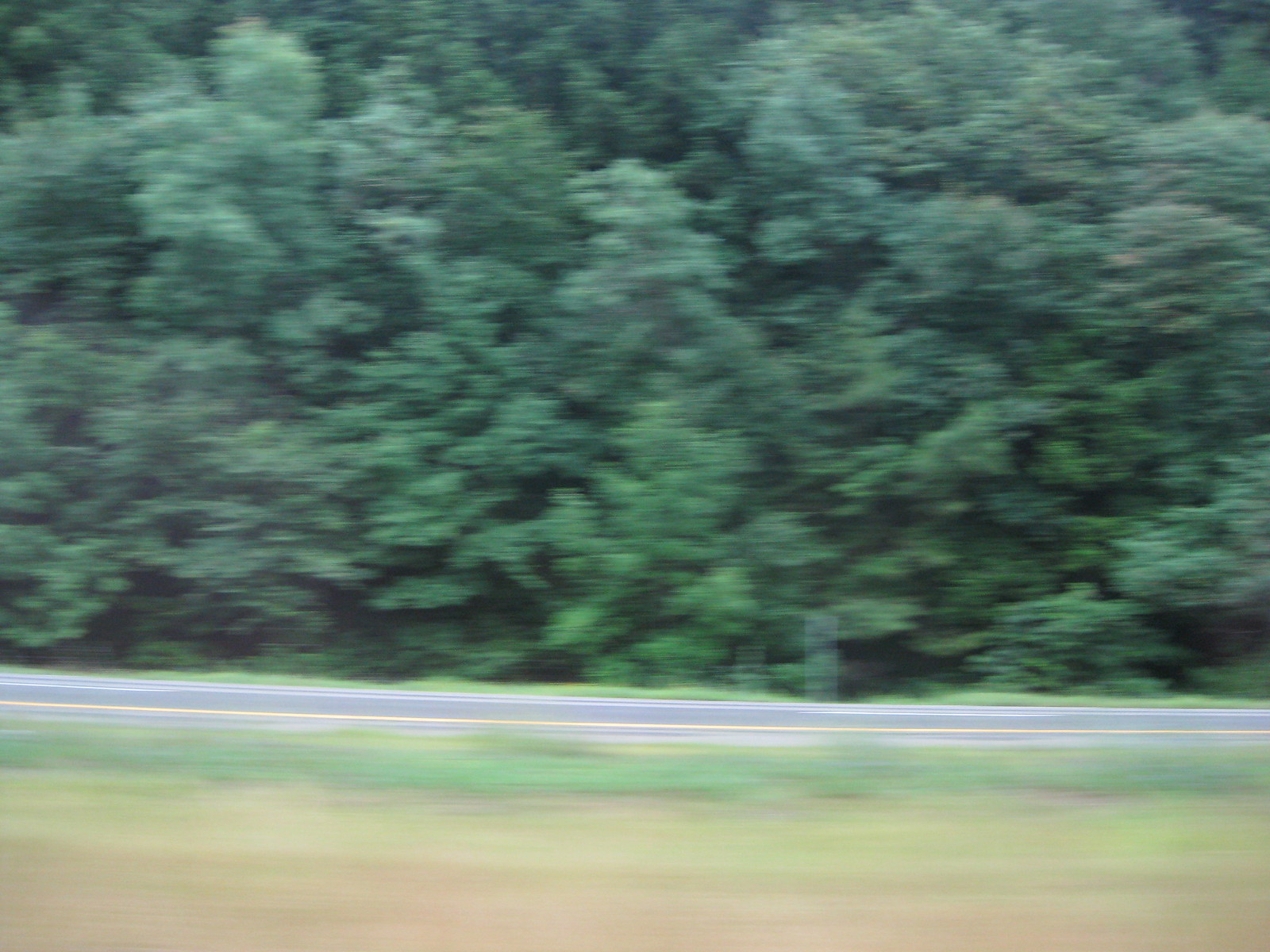A large, square photograph captures the view from the side window of a moving vehicle. The background is dominated by an impenetrable wall of dense, verdant trees, their branches thickly adorned with lush, green leaves. This dense foliage forms a continuous, green curtain that blocks any further view into the distance. In the middle ground, a patch of dirt transitions into a grassy area, leading up to a small road in the immediate foreground. The road, marked by a prominent yellow line, runs parallel to the dense forest, creating a striking contrast between the man-made and the natural elements in the scene.